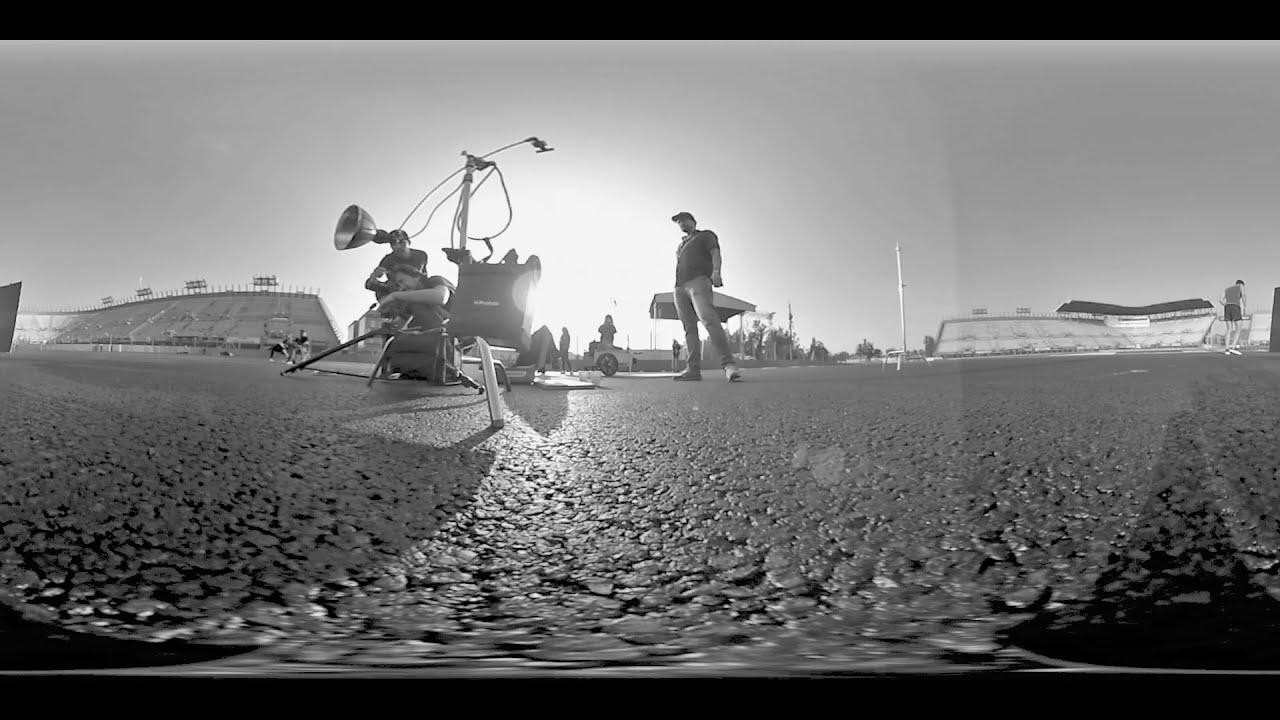This black-and-white photograph depicts an outdoor scene, possibly related to a sporting event or media production, in a parking lot or pebble-covered area. The landscape-oriented image features horizontal black stripes at the top and bottom. Prominently in the center stands a man wearing a baseball cap, dark shirt, and light pants, holding an object in his hand and appearing to be engaged with overhead microphone equipment. To the left, background structures include stadium stands with lighting fixtures resembling a moon lander due to their many parts and projections. The bright sunlight illuminates the area, reflecting off the textured ground, which looks like melting snow or wet stones. On the right, there's another set of stadium stands, and scattered throughout the scene are a few individuals, including another person crouched near some audio-visual equipment and a person standing with their back to the camera.